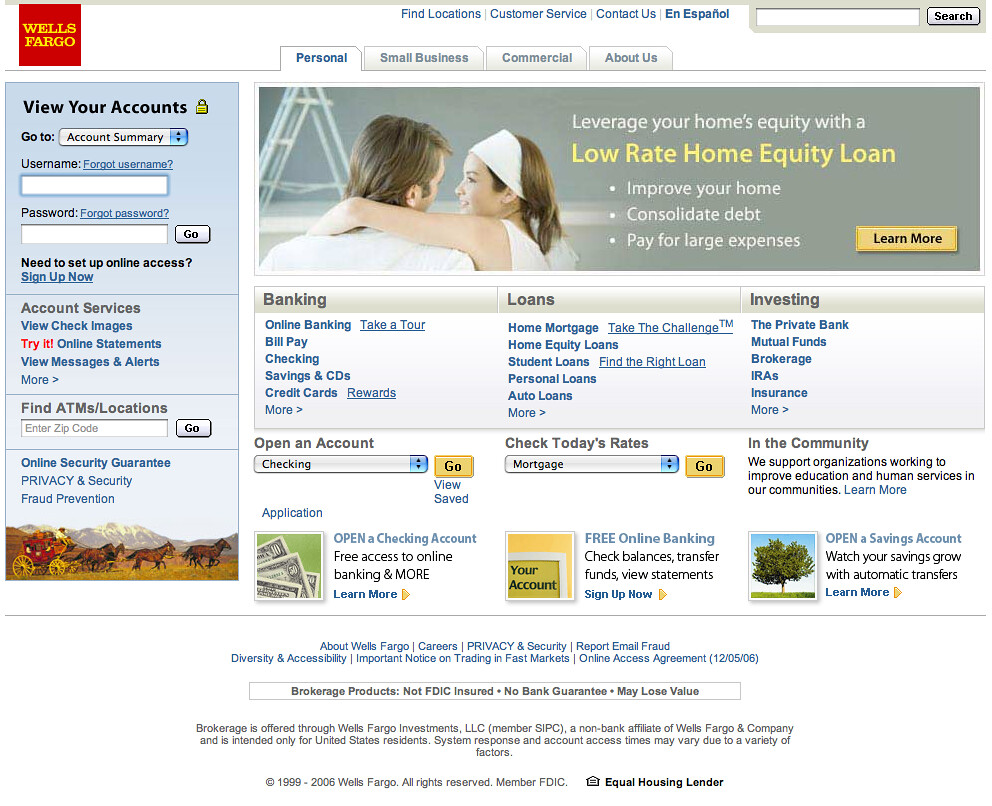The image is a detailed, left-to-right horizontal screenshot of a Wells Fargo web page, likely captured from a computer or smart device. The background prominently incorporates white space typical of a computer interface. At the very top, a long horizontal strip spans the width of the page, and in the upper left corner, the recognizable red square with the yellow Wells Fargo logo is conspicuously placed.

Towards the center of the strip, there are navigation links in blue text: "Find Locations," "Customer Service," "Contact Us," and "En Español." Adjacent to these options is a search bar with the placeholder text "search." Below the Wells Fargo logo, the text "View Your Account" appears, followed by a link to "Go to Account Summary." 

Below this, several interactive fields and buttons are visible for "Username," "Password," "Need to Set Up Online Access," and a "Sign Up Now" button. Additional sections labeled "Account Services" offer functionalities like "Check Images," "Try It," "Online Statements," "View Messages and Alerts," and more. The page also features a section to find ATMs and branch locations, where users can enter their zip code.

Further down, there is comprehensive information about "Online Security Guarantees," "Privacy," "Security," and "Fraud Prevention." A scenic image of mountains and horses pulling wagons is placed towards the bottom part of the page, adding a picturesque element.

At the top navigation bar, several tabs are displayed: "Personal" (highlighted), "Small Business," "Commercial," and "About Us." An advertisement depicting two people promotes leveraging home equity with a low-rate home equity loan. Additional details on banking, loans, investing, opening accounts, checking rates, and community information are also provided. Finally, standard footer links for privacy policies and other essential website elements are visible at the bottom of the page.